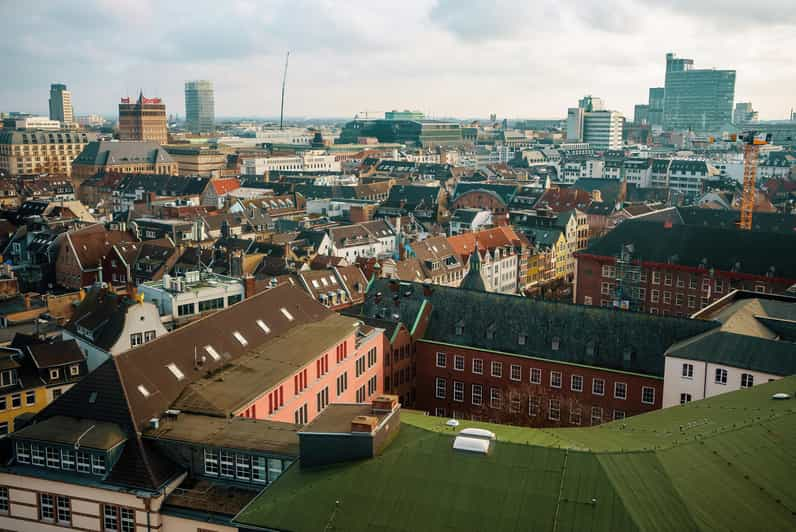This aerial photograph captures a densely packed European village or city with a predominantly dull and dingy color palette. Emphasizing the old-town feel, most of the buildings are constructed from brick or mortar, with light pink walls and dark red roofs prominently featured in the foreground. The varied architecture includes homes and apartment buildings that are closely situated, with heights generally around four to five stories. Among the sea of angled, brown rooftops, a distinctive building with a green roof stands out towards the right side of the image. The streets are narrow, and the spacing between the structures is minimal. Beyond the village, a few taller skyscrapers rise in the background, adding contrast to the otherwise uniform skyline. The sky above is overcast with gray clouds, contributing to the overall muted tone of the scene.